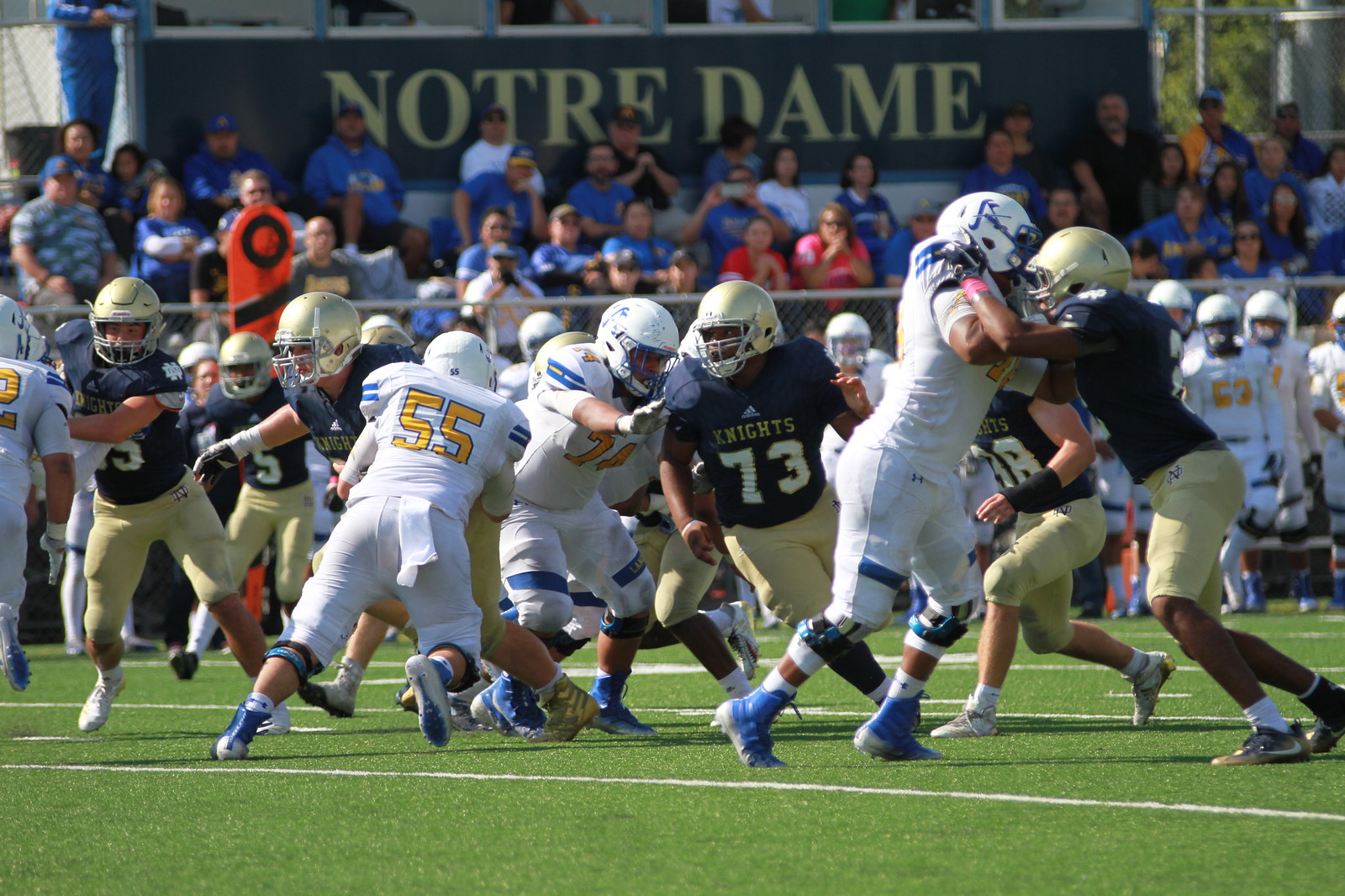In this professional-quality outdoor photo, we capture an intense football game on a pristine, green field marked with white lines. At the center of the action are the football players, specifically number 55, who is actively pushing against an opponent, and number 73, who is running towards the clash. The team with dark blue jerseys, gold helmets, and shorts, emblazoned with "Knights," represents Notre Dame. Their opponents sport white uniforms accented with medium blue stripes and yellow numbers. Behind the players, a vibrant crowd mostly dressed in blue and gold colors fills the stands. Above them, a prominent banner with "Notre Dame" in gold writing on a black background establishes the location. Notably, number 63 from the Knights is visible sitting on the bench, while the visiting team watches attentively from the sidelines.